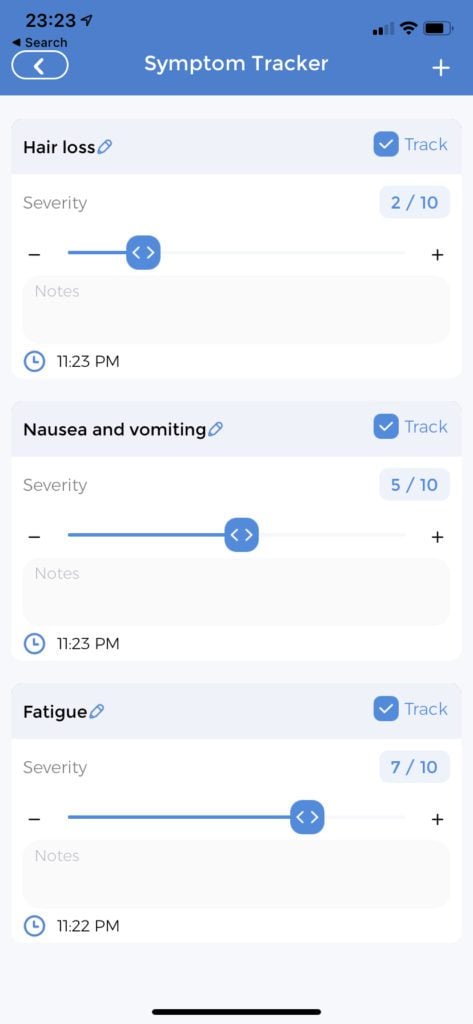This image is a screenshot from a cell phone displaying a symptom tracking application. At the very top, a blue header bar spans the width of the image. On the top left of this blue area, in black text, is the time "23:23". Positioned to the right of this time display are icons showing the signal strength bars, a Wi-Fi symbol, and a battery indicator.

Within the blue header area, centrally aligned and towards the bottom, is the title "Symptom Tracker." To the left of this title is an oval icon with an arrow pointing left, indicating a back function.

Below the blue header, the background transitions to a very light gray. This section is divided into three uniform blocks, each separated and outlined with a slightly darker gray border at the top of each block.

The first block is labeled "Hair Loss" on the left side. Next to this label is a blue checkbox marked "Track". Underneath, a subheading "Severity" is accompanied by a horizontal slider bar, indicating a measured severity level of 2 out of 10. Below this, a section for notes is symbolized by a small clock icon followed by the time "11:23 p.m."

The second block follows the same structure but is labeled "Nausea and Vomiting". Here, the severity level is set to 5 out of 10, with the same note and the timestamp "11:23 p.m."

The third and final block is titled "Fatigue". Its severity level is marked as 7 out of 10, and the timestamp for the notes is "11:22 p.m."

Each block maintains consistency in format: the left-aligned title, a checkbox for tracking, a severity slider, and a timestamped notes section.